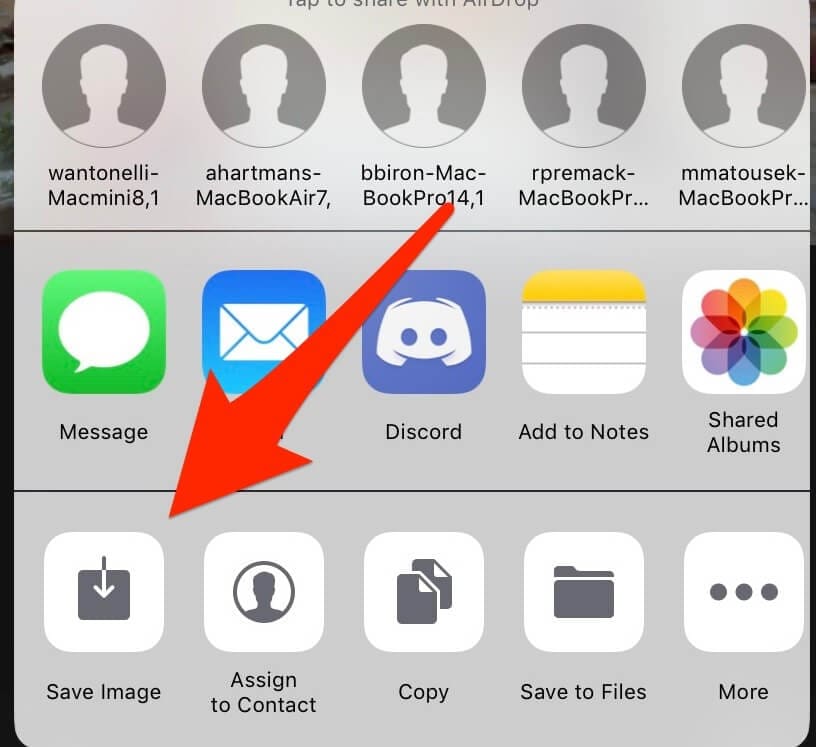The image shows a close-up view of a phone screen with a predominantly gray background. The screen is divided into three distinct sections with the left and right corners fading into black. 

At the bottom of the screen, there are five clickable tabs, each inside a gray square. From left to right, they are labeled:
1. "Save Image"
2. "Assign to Contact"
3. "Copy"
4. "Save to Files"
5. "More" (depicted with three gray circles).

A red line extends from the first row at the top, starting at the label “BBIRLND-MAC-BOOK-PRO-14,” and points towards the "Save Image" tab.

The second row features four app icons:
1. A green icon labeled "Messages"
2. A blue icon partially obscured by an arrow, possibly labeled "Mail."
3. A different blue icon labeled "Discord."
4. A yellow, white, and black icon labeled "Add to Notes."
5. A multicolored icon labeled "Shared Album."

Above these app icons are five light gray circles containing the image of a person, indicating five contacts. The contact in the middle is highlighted with a red arrow. The contacts at the bottom are optionally labeled as:
- "MAC Mini 8-1"
- "MAC Book Air 7"
- "BBIRLND-MAC-BOOK-PRO-14" (corresponding to the red line)
- "MAC Book PR..." (partially obscured).